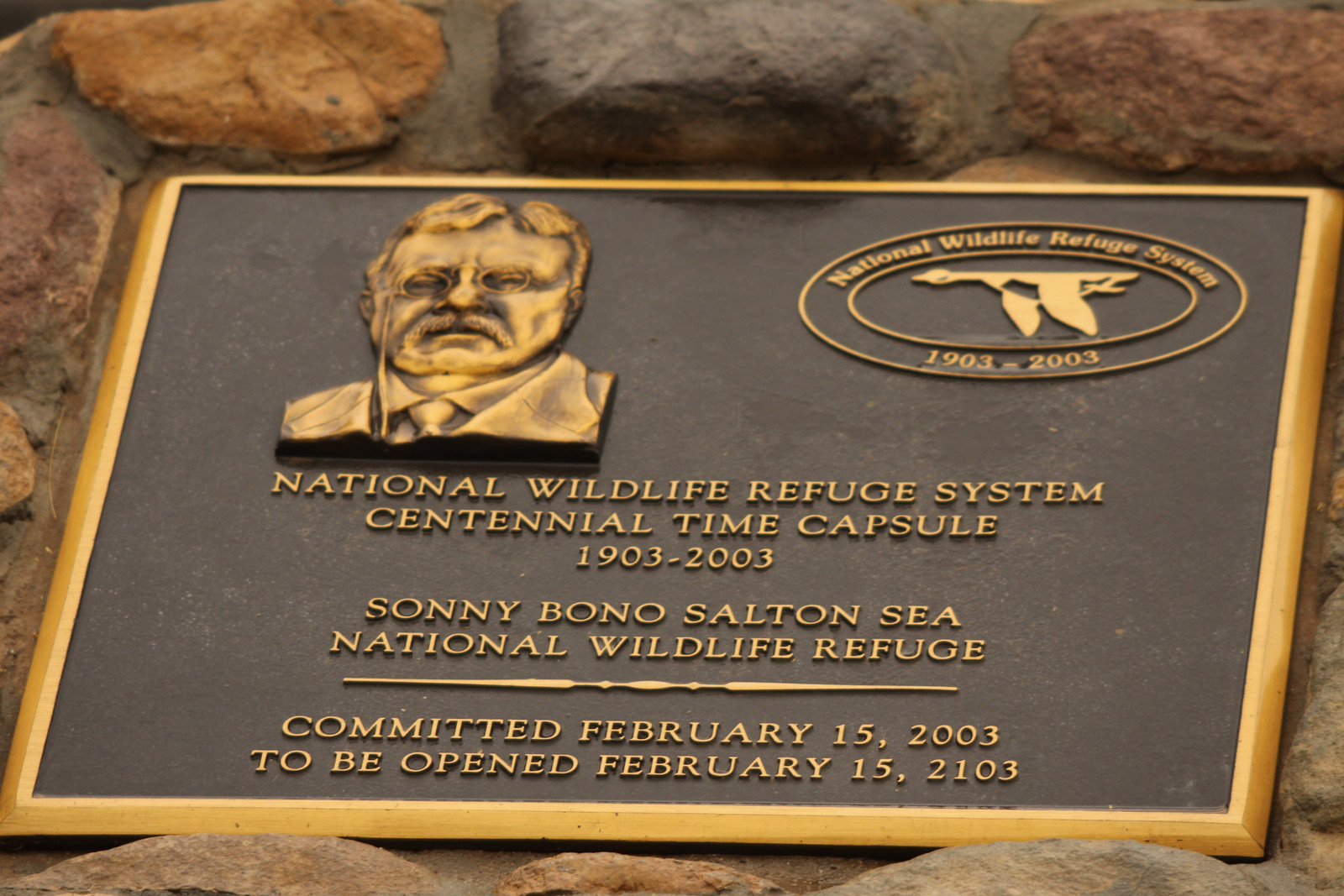The photograph shows a detailed, rectangular plaque embedded into a stone podium outdoors, surrounded by large, mortared stone boulders of various shapes and colors. The plaque is slightly tilted upwards. It features a beveled gold border and a black background. In the upper left-hand corner, there is a raised golden bust of Theodore Roosevelt, recognizable by his signature eyeglasses and mustache, depicting him from the shoulders up. To the right of the bust, there is an emblem with an outer and inner oval. The outer ring of the emblem reads "National Wildlife Refuge System" at the top and "1903-2003" at the bottom, while the inner oval contains a flying goose.

Below the emblem and bust, gold-raised lettering on the plaque reads: "National Wildlife Refuge System Centennial Time Capsule, 1903-2003, Sonny Bono Salton Sea National Wildlife Refuge." A horizontal line separates this text from the succeeding inscription: "Committed February 15, 2003, to be opened February 15, 2103."